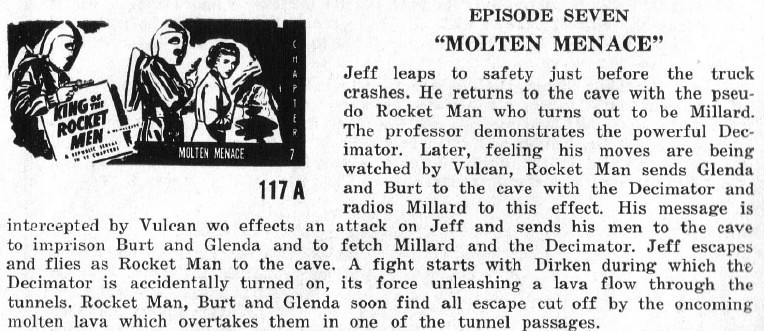The image is an old book clipping featuring Chapter 7, titled "Molten Menace," from the serialized story "King of the Rocket Men." On the left-hand side, there is an illustration showing two masked men, likely equipped with jetpacks, and a woman. The masked men appear to be Rocket Man with rocket packs allowing them to fly.

The text, wrapping around the illustration, describes a dramatic scene where Jep narrowly escapes a truck crash and heads back to a cave as Rocket Man. The chapter escalates with Rocket Man, Bert, and Glenda trapped in a cave as molten lava flows through the tunnels following an altercation with Durkin. The passage reveals that Rocket Man's actions are under surveillance by Vulcan, who sends his men to capture Bert and Glenda and seize a powerful device called the decimator. Despite their efforts to escape, the characters find themselves surrounded by the advancing lava in the cave's tunnels, highlighting the perilous situation they face. 

This clipping not only provides a glimpse into the adventurous and hazardous world of Rocket Man but also captures the vintage essence of storytelling from possibly the mid-20th century.